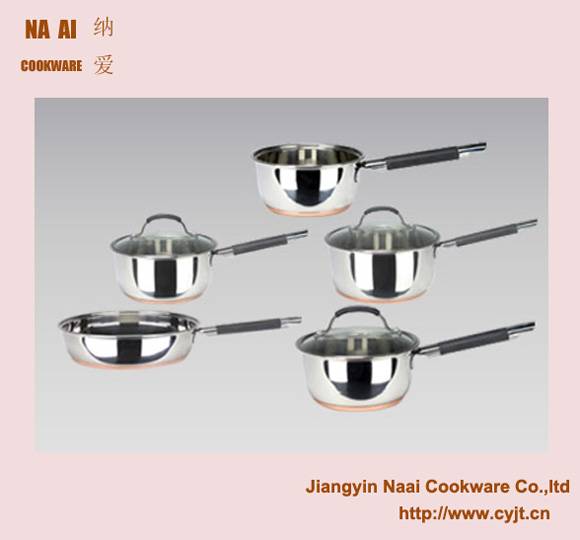This is an advertisement for Jianjin Nai Cookware Company Ltd., featuring their collection of copper-bottom pots with silver finishes. The image showcases a total of five pieces, including various-sized saucepans, pots, and a skillet, with three of these having lids. Each piece is equipped with handles, suggesting practical design and usage. The advertisement has a light pink border, and the background is gray. In the top left-hand corner, "NAAI Cookware" is prominently displayed, possibly accompanied by Chinese symbols. The bottom right corner features the full company name, Jianjin Nai Cookware Company Ltd. (C-O-L-T-D), along with their website, www.cyjt.cn.